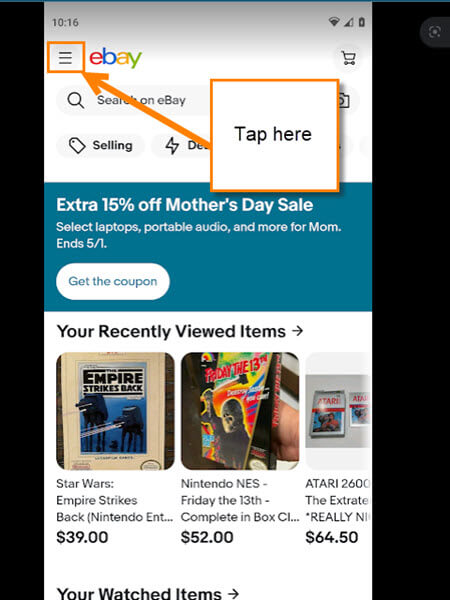The image is a vertically oriented screenshot of a cell phone screen with black letterboxing on the right and left sides, occupying roughly 20% on the right and 10% on the left. The cell phone screen displays what appears to be the eBay app or website. At the very top, the screen shows a white background with black text displaying the time "10:16" on the upper left. On the upper right, icons indicating Wi-Fi, wireless signal, and battery life are visible.

Below the status bar, on the left-hand side, there is a notable feature – the eBay menu. This prominently includes the eBay logo situated next to three vertically aligned horizontal lines, forming a classic menu icon. An orange square overlays the menu area, drawing attention to it. An arrow extends from the right side of this square, leading to another orange box on the far end. The second box contains the black text "Tap here," indicating an interaction cue aimed at guiding the user to the menu.

Beneath this highlighted section lies typical eBay interface elements including a search bar and several buttons. Additionally, there is a section displaying recently viewed items, further cementing the context of the app in use. The meticulous visual indicators and clear labeling within the image effectively guide the user on how to navigate the menu within the eBay app.